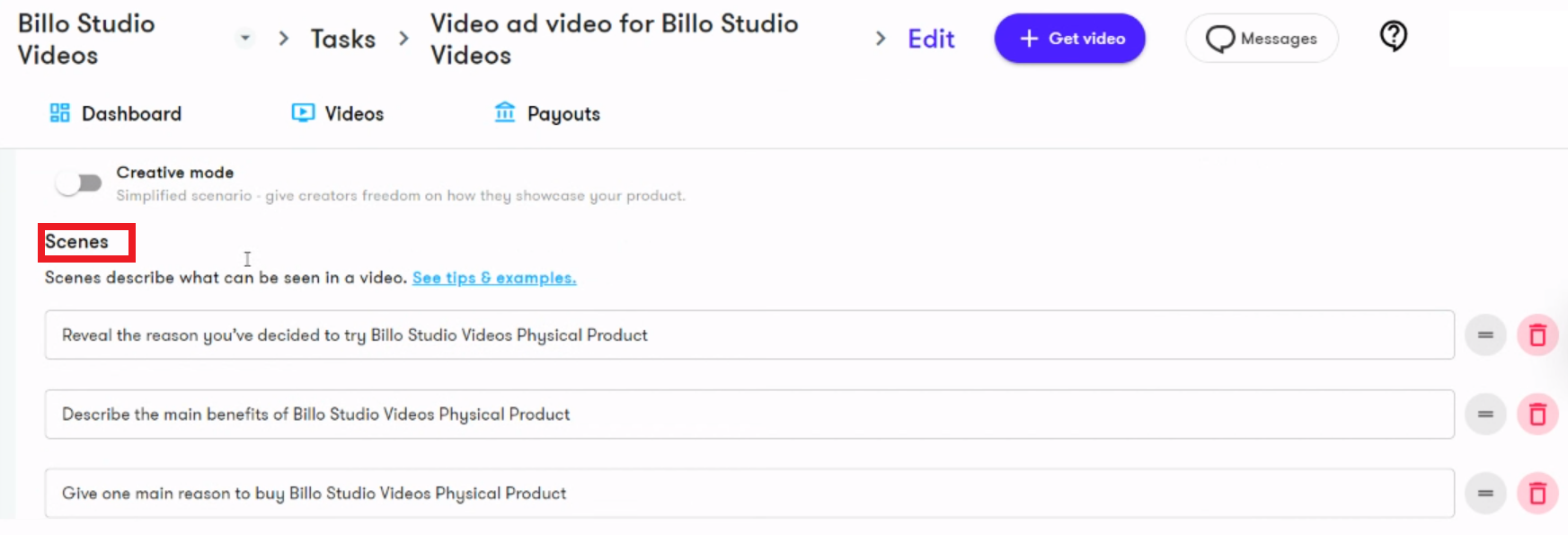A screenshot of a website interface is captured. The top-left corner of the image features a breadcrumb trail indicating the user's navigation path, starting from "studio videos." Following the trail, arrows guide the sequence: "studio videos" → "tasks" → "video" → "add video" → "edit." Adjacent to the "edit" tab is a prominent purple, horizontally-oriented oval button labeled "Get Video." To its right, there is a "Messages" button, followed by a question mark icon within a speech bubble, suggesting a help or FAQ feature.

Directly below this navigation section, three tabs with blue logos are aligned horizontally: "Dashboard," "Videos," and "Payouts." Below these, options for "Creative Mode" and "Scenes" are listed, with "Scenes" highlighted by a red rectangle, possibly denoting its active status or importance.

Further down, explanatory text provides guidance on content creation for Below Studio's physical product. It reads: 
- "Scenes describe what can be seen in a video."
- "Reveal the reason why you've decided to try Below Studio Videos physical product."
- "Describe the main benefits of Below Studio's physical product."
- "Give one main reason to buy Below Studio's physical product."

This suggests that the website content serves as an instructional guide for creating promotional material for Below Studio’s product, outlining key points that should be addressed in the advertisement.